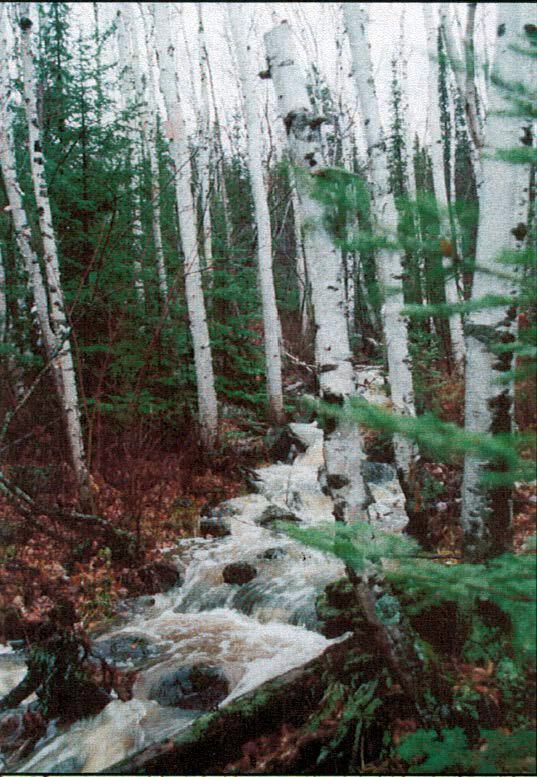A striking vertical photograph captures a forest landscape, featuring tall trees with white bark, some as thick as torsos, others as slender as arms, adorned with green leaves. The ground is carpeted in a mix of brown and tan leaves, indicative of autumn or early winter. An eight-foot-wide stream, resembling a miniature white-water river, roars through the center of the scene, its waters crashing over approximately 20-pound rocks and creating frothy white waves. Slender trees and bushes with green foliage intermingle with the taller, white-barked trees, while the pale overcast sky peeks through the canopy above, casting a subdued light over the predominantly white, green, and brown landscape.